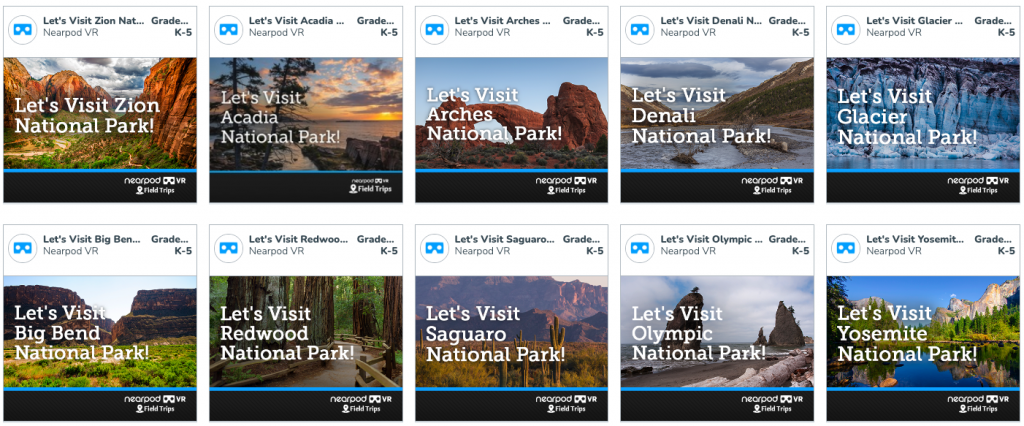This image is a screenshot from a website, likely for a travel agency or an educational platform, showcasing virtual reality tours of various national parks. The image is rectangular and horizontally oriented. It features two rows of five boxes each, displaying different national parks.

In the upper left corner of the image, there is a photograph of orangey-colored mountains with clouds, grass, and trees. Overlaid at the top, it says "Let's visit Zion National Park," and beneath that, "Grade K to 5 Nearpod VR." Each box in the image has a small VR symbol in the upper left corner, depicting blue virtual reality glasses.

Adjacent to this, another box displays an image of water, boulders, trees, and a sunset with white clouds. It is labeled "Let's visit Acadia National Park," with similar text noting "Grade K to 5 Nearpod VR."

These boxes appear to be part of a website that offers virtual reality experiences for visiting national parks, specifically designed for students from Kindergarten to 5th grade.